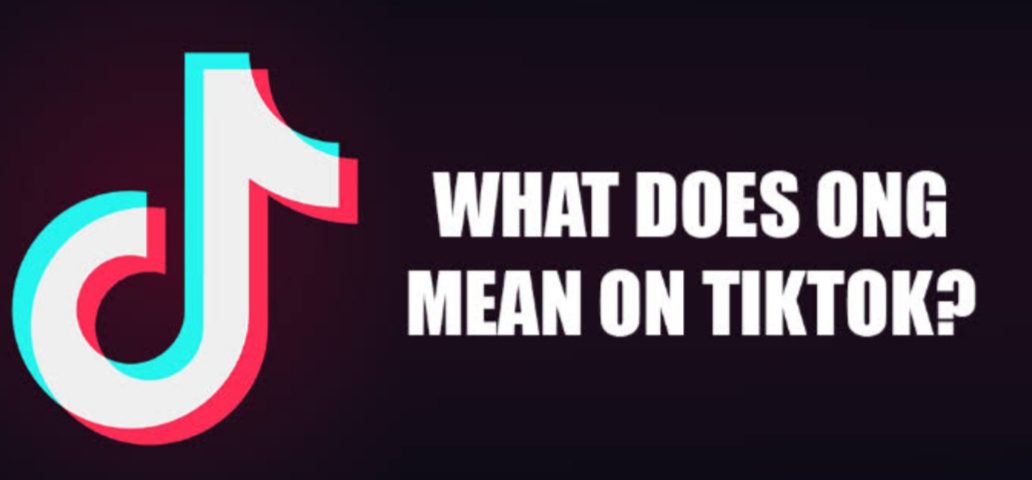The image features a rectangular black background with large, bold white lettering that reads, "What does O-N-G mean on TikTok?" On the left side of the text is a stylized icon resembling the TikTok logo, which is designed with a lowercase "d" shape. This logo has a white center, a blue outline, and a red inline, giving it a distinctive and colorful appearance. The entire composition is focused on the central question, providing a visually straightforward yet striking layout aimed at drawing attention to the query about the meaning of "O-N-G" on the TikTok platform.